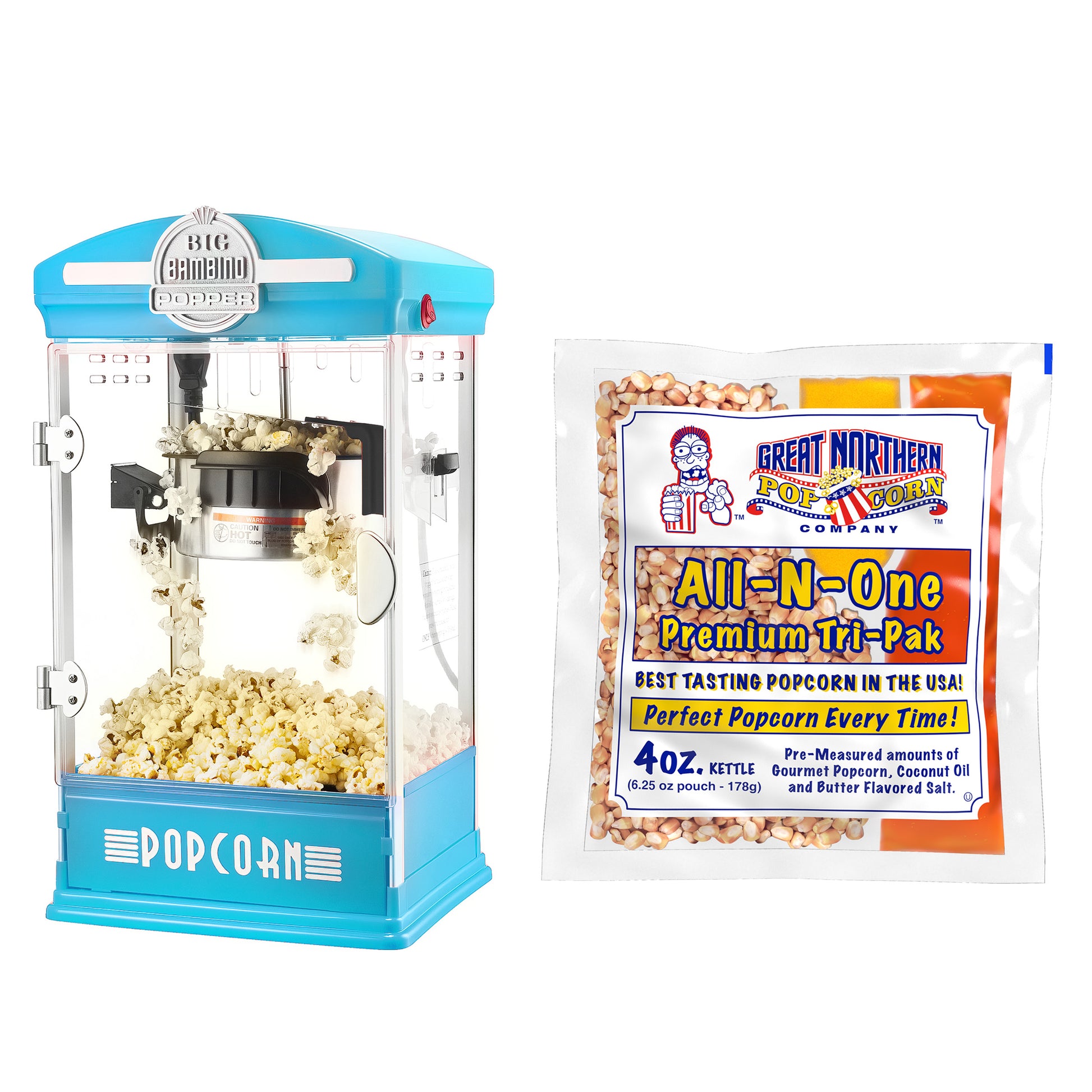In the image, there is a small tabletop popcorn maker positioned on the left side, featuring a distinctive light blue tin base and top. The base is labeled "Popcorn," flanked by white lines on both sides of the word, and prominently displays an emblem at the top that reads "Big Bambino Popper." Inside its glass windows, bright yellow popcorn is actively popping, providing a clear view of the popcorn-making process.

To the right of the popcorn maker, there is a clear package of popcorn kernels from the Great Northern Popcorn Company, labeled as "All-In-One Premium Tri-Pack." The packaging includes multiple inscriptions: "Best Tasting Popcorn in the USA," "Perfect Popcorn Every Time," "4oz Kettle," "Pre-Measured Amounts of Gourmet Popcorn," "Coconut Oil," and "Butter Flavored Salt." The background of the image is solid white, focusing all attention on the popcorn maker and the accompanying packaging.